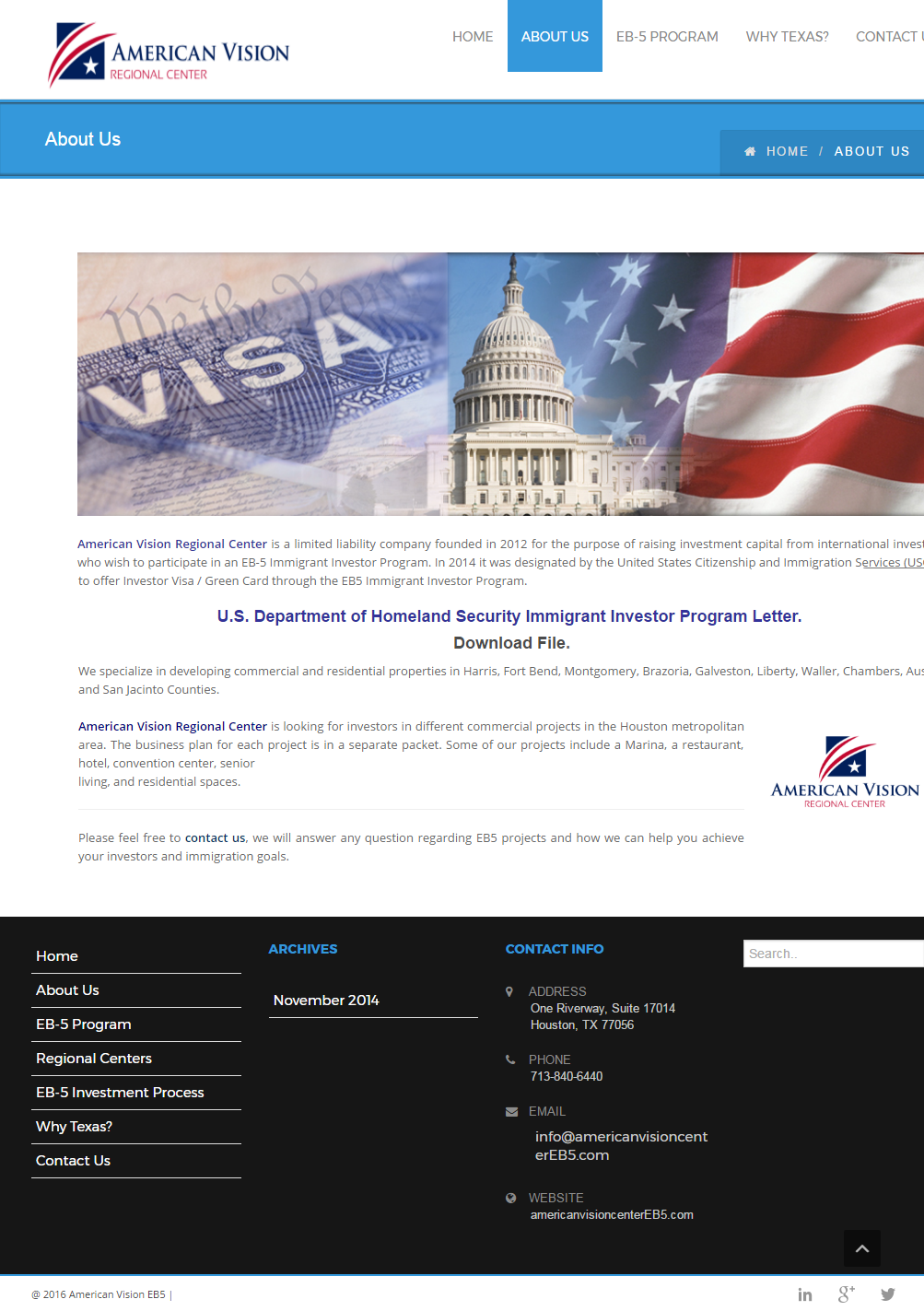The image features a white border at the top, followed by the logo and name "American Vision Regional Center," which is represented with a red, white, and blue star icon. To the right, the header navigation includes the options "Home," "About Us" (highlighted with a blue box), an unreadable smaller text presumably for a program, "Why Texas," and "Contact." Below the navigation, a blue header repeats the options "About Us," "Home," "About Us."

The main section of the image displays a composite featuring the Declaration of Independence overlaid with a visa, along with the Capitol building in Washington, D.C., and an American flag to the right. Beneath the image, there is a paragraph of text that is too small to read. Further down, a link states "US Department of Homeland Security Immigrant Investor Program letter download file." Additional unreadable text follows, and at the bottom, a black footer contains links to "Home," "About Us," a program section, "Regional Centers," and something related to the investment process.